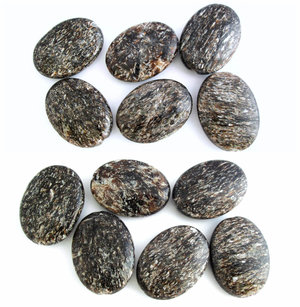The image depicts 12 polished, oval-shaped cabochons, likely made of jasper, resting on a plain white background with subtle shadows. These stones are uniformly smooth and rounded, suggesting they might be good for skipping. The stones are organized into two uneven groups of six, with the top group arranged symmetrically while the bottom group displays a more random alignment, including two horizontally positioned stones. Each cabochon exhibits a predominantly dark color with a mixture of beige, light brown, and black, along with specks of rust and warm sepia tones creating a stripy yet broken pattern across their surfaces.